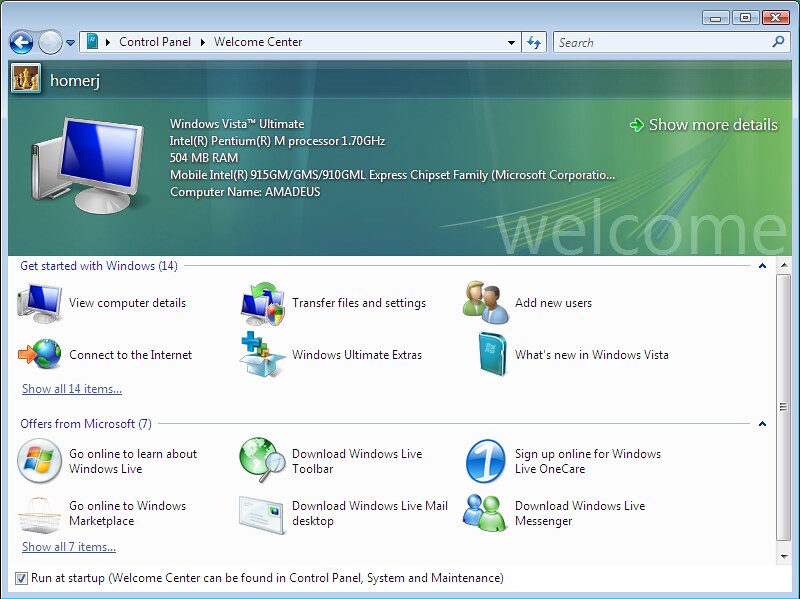The image is a detailed screenshot of a Windows Vista Ultimate Welcome Center from a Windows-based computer, likely a Windows Vista system. In the top left corner, it displays a user profile with the username "HomerJ" and a profile picture of a chess piece. The control panel window has light blue edges and borders, with "Welcome Center" written at the top alongside a search bar. Below this section, system specifications are listed: Windows Vista Ultimate, Intel Pentium M processor, 1.70 GHz, 504 MB RAM, and a Mobile Intel 915 GM/GMS, 910 GML Express chipset family. 

Further down, multiple icons represent various startup and getting started items, such as Transfer Files and Settings (with a file icon), Add New Users (depicted by two people icons), Connect to the Internet (globe icon), Windows Ultimate Extras, What's New in Windows Vista, and more. Additional options visible include viewing computer details and multiple online resources, such as downloading Windows Live Mail Desktop or signing up online for Windows Live OneCare. The Welcome Center screen indicates it will run at startup, controlled by a checkbox option, and is also accessible via the Control Panel under System and Maintenance.